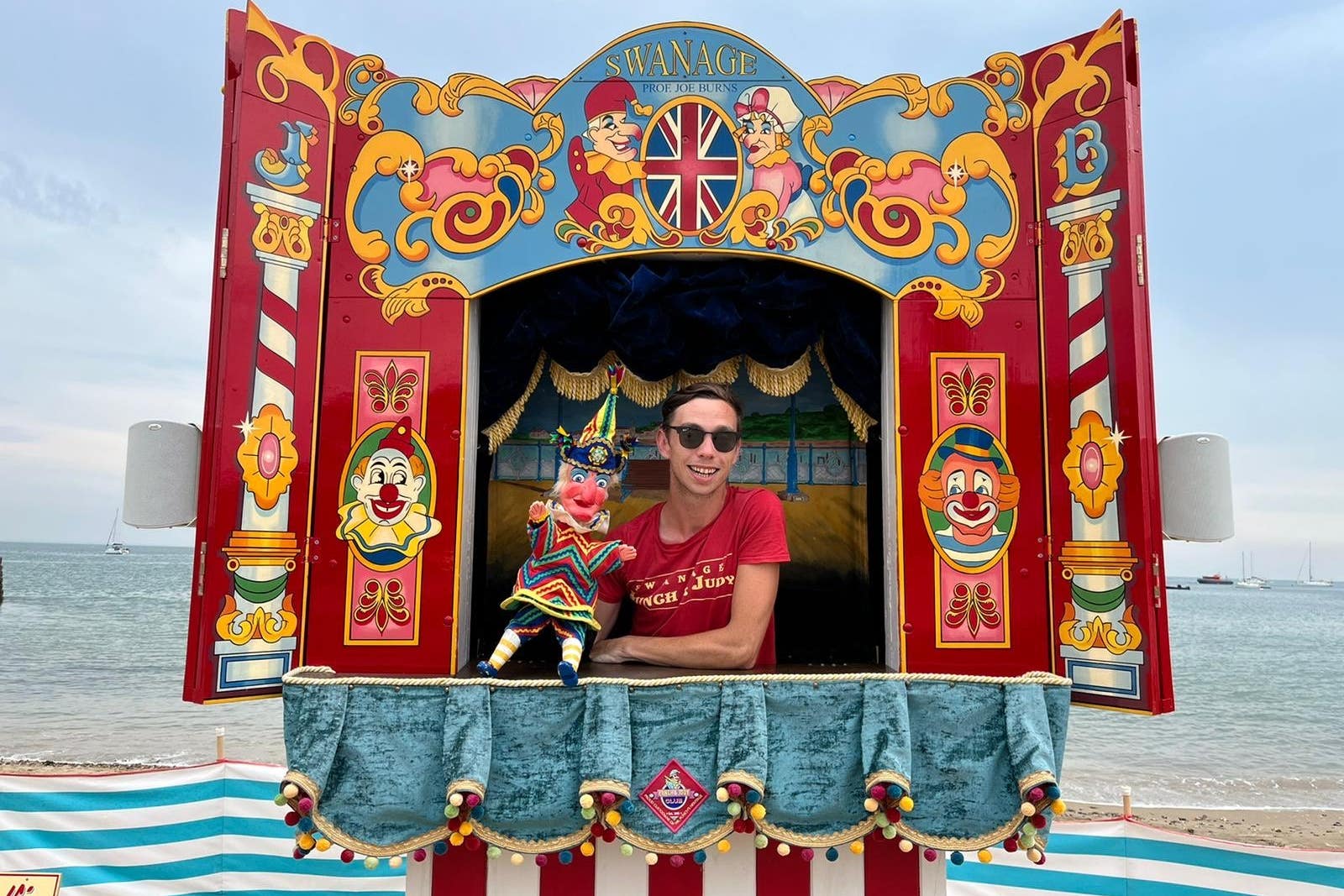This vibrant seaside photograph captures a lively puppet show taking place on a sunny day at the beach, with the ocean and sailboats visible in the background. The puppet theatre, adorned with bright and colorful clowns illustrated on red and white striped pillars, features a white and blue striped tarp acting as a fence. At the top of the stage, a sign reads "Swanage, Professor Joe Burns," with the British flag waving cheerfully. 

In the center, a cheerful young man, possibly in his early 20s, stands behind a red podium draped in rich blue velvet and pleated fabric. He wears a red T-shirt emblazoned with "Swanage" and "Punch and Judy" in white text, along with sunglasses and a smile that matches the lively atmosphere. The man masterfully holds a puppet representing either Punch from "Punch and Judy" or an old lady with a colorful, rainbow-colored hat and multicolored clothing. The puppet's bright red face and vibrant attire add to the joyful scene.

The puppet stage itself is intricately designed with blue pleats and golden cord-draped curtains framing the sides. The colorful drawings, which include depictions of swooshes and decorative details in an array of blues, golds, pinks, oranges, and more, add to the overall merry ambiance of this seaside puppet show.